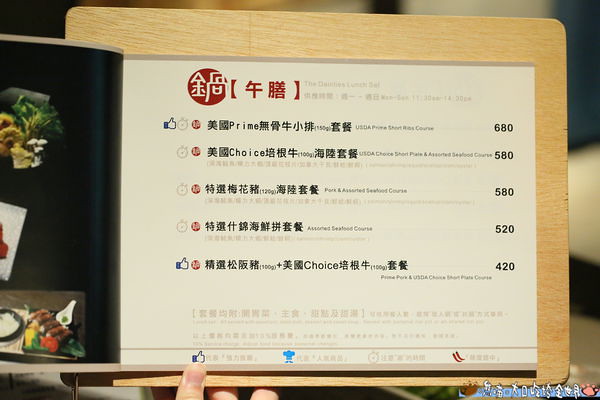The image depicts a detailed restaurant menu attached to a wooden board, likely situated in an Asian country, suggested by the use of Chinese characters. The top section of the cream-colored paper menu features a red logo with Chinese characters, and underneath that is partially visible grey text, potentially reading "Lunch Special." The menu lists several dishes in both Chinese characters and English. The English text reads "USDA prime short rib course 680," followed by "Choice USDA choice short rib and assorted seafood course 580," "Pork and assorted seafood course 580," "Assorted seafood course 520," and "Choice prime pork and USDA choice short rib course 420." These dishes are accompanied by corresponding prices in black and maroon colors. Additionally, a hand is visible at the bottom of the image, with a finger pointing to the menu. On the left side of the board, there appears to be another menu page with pictures of the food served, giving a visual representation of the offerings.